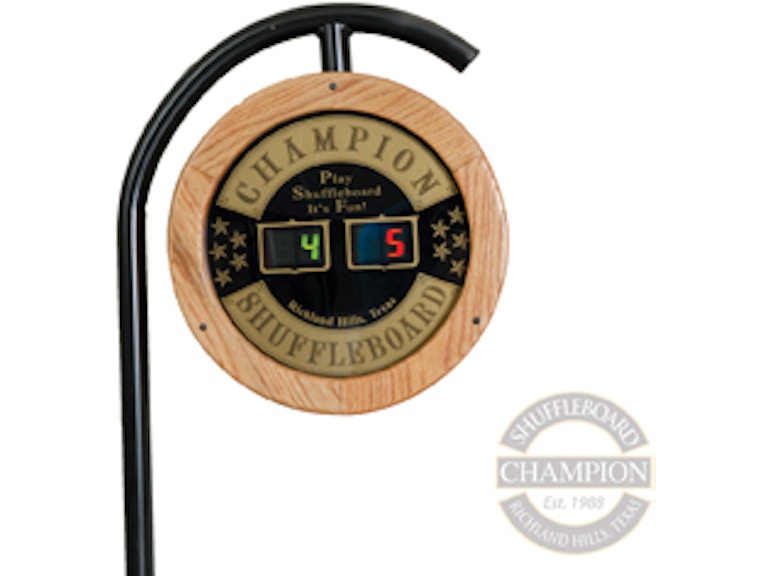This image showcases a stylized design of a champion's medal. On the left side, a vertical black holder, reminiscent of a candy cane shape, curves to the right before dropping down. Attached to this holder is the medal, which features a light brown outer edge. The word "Champion" is prominently displayed in brown text against a faded gold background. Below this, the word "Shuffleboard" is also written in brown text on the same gold background. On either side of the medal, there is a black strip adorned with five gold stars. At the top of the medal, in very small text, the left side reads "4" in green, and the right side reads "5" in red. The center of the medal showcases a white background with an emblem that states "Shuffleboard Champion EST 1963" accompanied by additional text, all in gray.